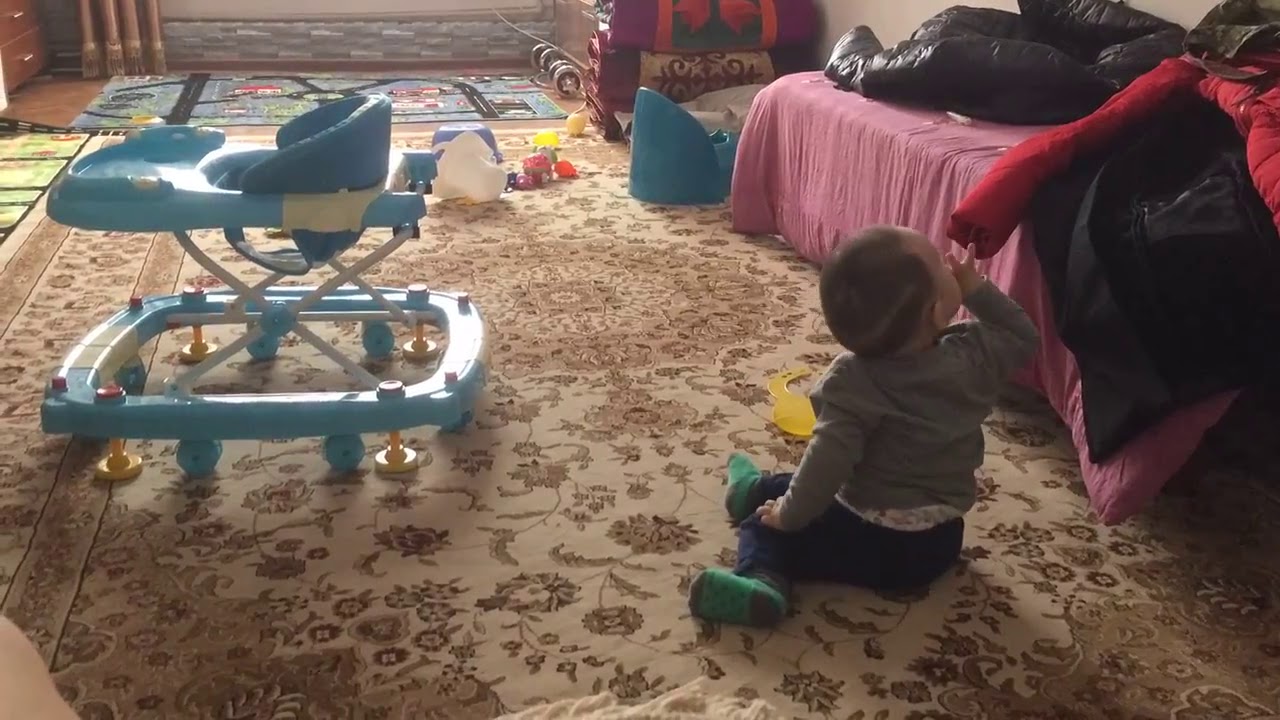The image depicts a children's playroom with a toddler, around two years old, sitting on a tan and red floral area rug. The child, dressed in a gray sweater, plaid shirt, blue pants, and green socks, is carefully touching the sleeve of a red down jacket that lies on top of a spread-covered couch or bed. The sunlight filters through a nearby window, casting a warm glow over the scene. Next to the child, there is a blue and white walker with yellow feet, equipped with six wheels. Scattered around the floor, there are various children's toys, including a yellow ball and a tan ball. In the background, on the right side, there's a blue chair. The scene is cozy and inviting, focusing on the child who seems intrigued by their surroundings.